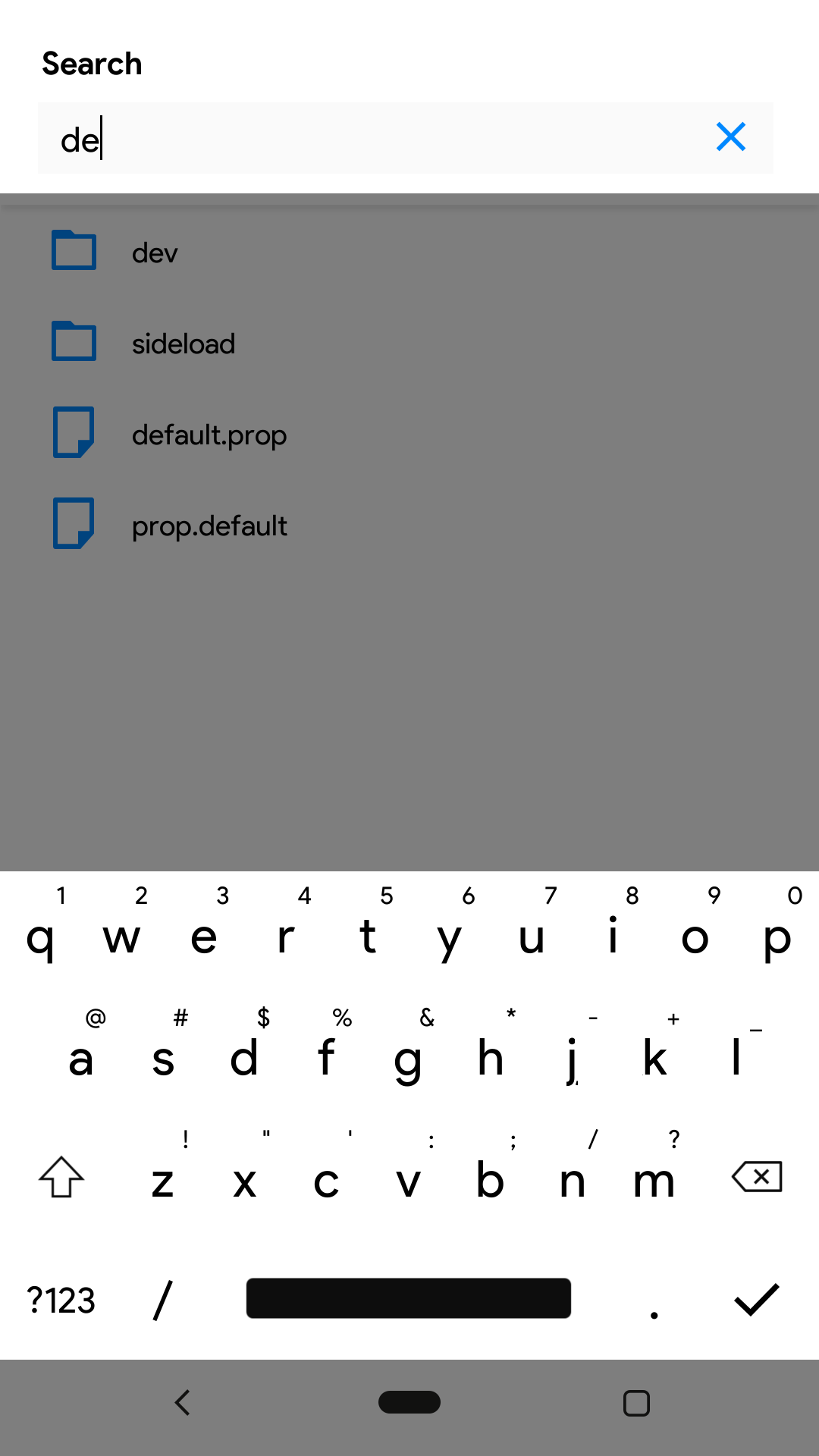In the image, the top section features a search bar labeled "Search." Inside the search box, the text "DE" is visible, with a blue 'X' button on the right side. Below the search bar is a dark gray area containing two blue folder icons labeled "DEV" and "SIDELOAD." Additionally, there are two file icons named "DEFAULT.PROP" and "PROP.DEFAULT."

Beneath this gray section is a keyboard displayed against a white background. The keyboard layout includes keys arranged from top left to bottom right with the letters "QWERTYUIOPASDSGHJKLDXCVBNM." Other keys visible on the keyboard are the Backspace key, the "1-2-3" key, a question mark key (/), the space bar, and a check mark key for confirmation. Below the keyboard lies a gray box area.